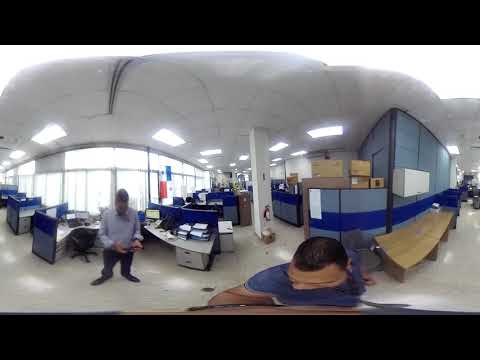The image appears to be a 360-degree shot taken from within an office building, rendered with a heavily warped, fisheye-like effect that causes everything to appear rounded and distorted. The environment is bathed in daylight, contributing to the clarity of the details. Dominating the bottom center of the image is the photographer, a person with brown skin, dark brown hair, and wearing a short-sleeved dark blue shirt, who is looking down at possibly a phone. Their arm is visibly extended in a distorted manner due to the lens effect.

To the left of the photographer stands another individual in a light blue shirt and dark pants, appearing shorter than normal because of the camera's distortion. They are positioned in front of blue and white office cubicles that look unusually rounded and compact. This section of the office also features a row of desks aligned beside a glass wall that opens to an outdoor space.

Further back in the image, towards the center-right, there is a hallway leading deeper into the office. This hallway is flanked on one side by a blue wall with stripes and a curve, featuring brown benches that appear similarly distorted. Additionally, a white column and ceiling lights are visible, contributing to the structured feel of the space.

Overall, the photograph captures a dynamic and somewhat surreal view of a modern office environment, blending stretched and rounded elements with both clarity and a touch of whimsy.